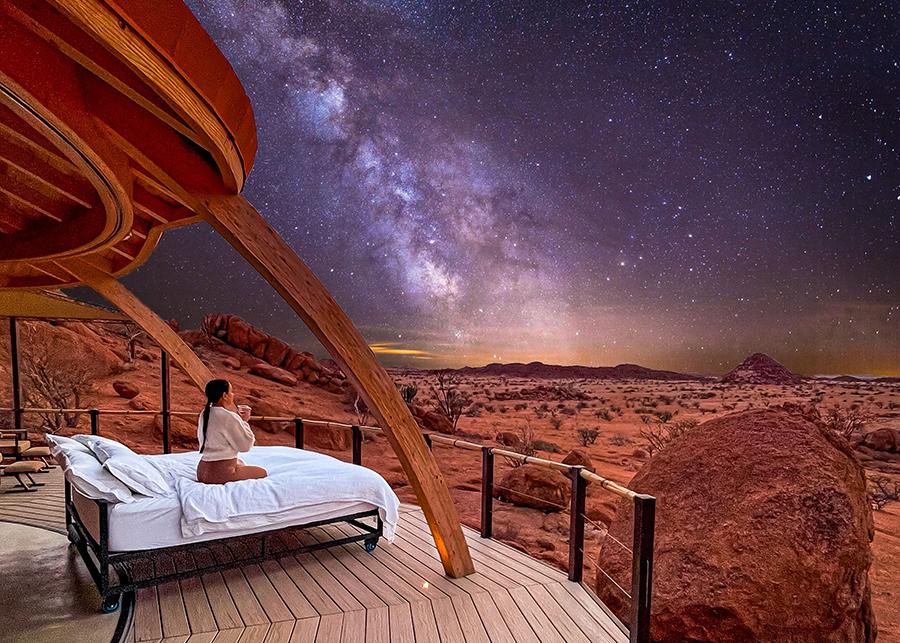The image portrays a surreal nighttime scene blending elements of realism and fantasy. Situated in the bottom left corner is a circular wooden patio with a guardrail composed of three wires. The patio houses a minimalist bed with a black frame and white bedding, including a comforter and two pillows. A woman, dressed in a light tan shirt and brown pants, sits cross-legged in the center of the bed. She has dark hair intricately braided down to her waist, and she is holding a mug.

The scene around the patio transitions into a stark, Mars-like desert landscape characterized by vibrant reddish-brown hues, large boulders, and sparse plant life. In the distance, the desert is framed by majestic red mountains, resembling the iconic rock formations of Sedona, Arizona.

Above the scene, an awe-inspiring night sky unfolds in stunning detail, filled with an array of stars and the luminous streaks of the Milky Way. The sky features a mesmerizing palette of purples, blues, and touches of yellow near the horizon, creating an otherworldly atmosphere. The intricate details and striking contrasts between the serene, intimate setting on the patio and the expansive, dramatic desert and celestial elements combine to create a powerful visual narrative.